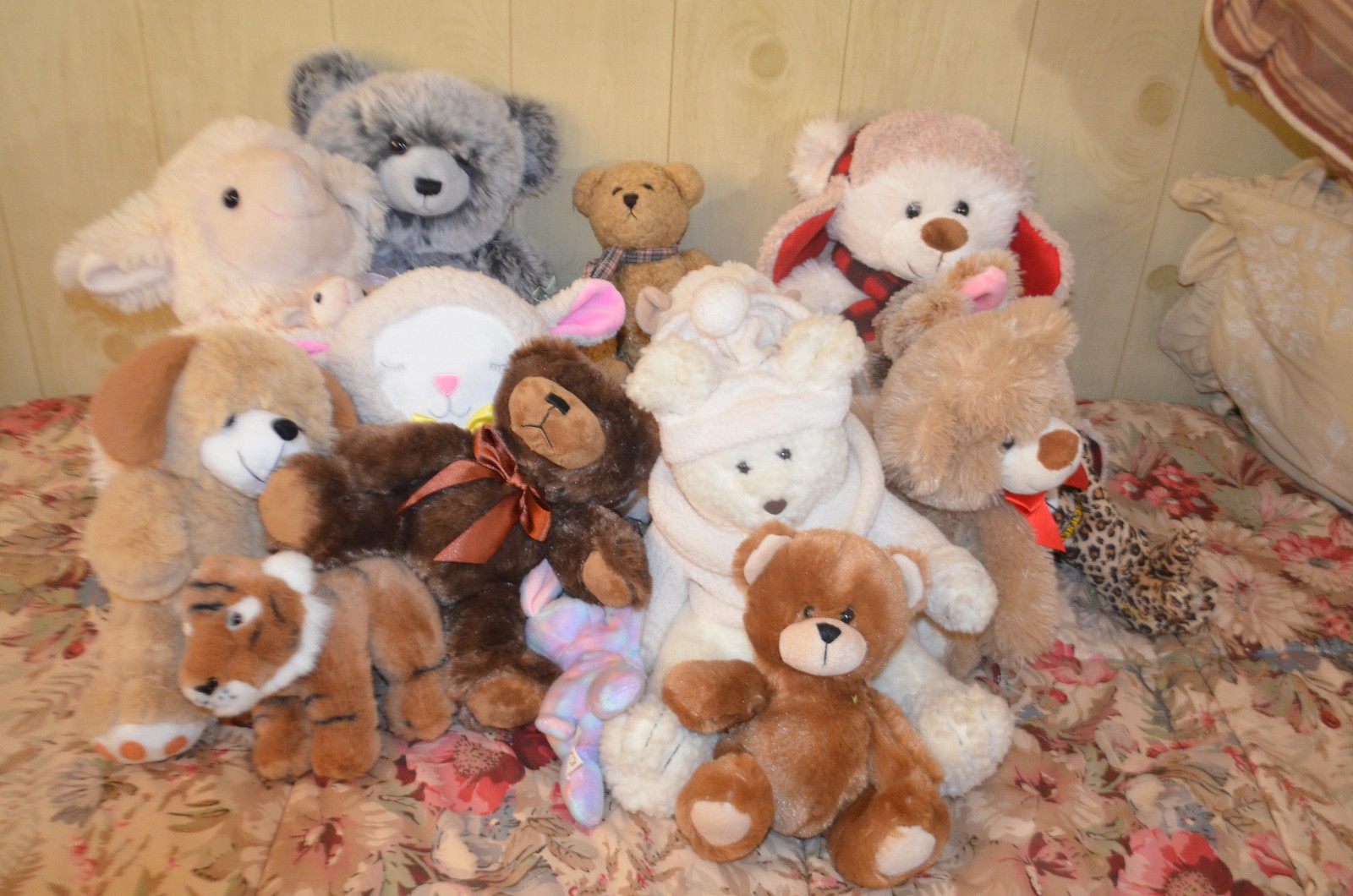The photograph captures a cozy and nostalgic scene: a bed adorned with a vintage tan bedspread featuring a busy floral pattern in red, burgundy, and blue hues. The bed is placed against a vertically paneled wall made of light, knotty blonde wood, further enhancing the antique rustic charm. A collection of approximately 12 to 15 stuffed animals is carefully arranged on the bed, creating a sense of cherished companionship.

Among the stuffed animals, there are several teddy bears of varying shades and sizes, including a dark brown teddy bear with a red bow, a smaller brown bear, a white teddy bear with a hat, and a tan bear with a checkered muffler. A notably large gray bear stands at the back, while a fluffy, off-white lamb with pink ears also finds a spot in the lineup. Additionally, a small stuffed Bengal tiger with striking stripes and a little dog with long brown droopy ears add variety to the plush ensemble.

The stuffed animals are tightly packed, facing forward as if posed for a group photo, each one adding its own unique charm to the arrangement. The bedspread's floral motif and the frilly pillow sham in the background contribute to the warm, welcoming feel of the scene. The soft, dull interior lighting casts a yellowish hue over the setting, evoking a sense of nostalgia and comfort from a bygone era.